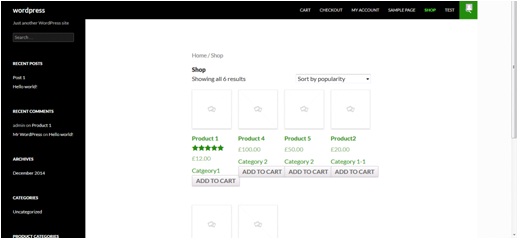This image is a small, low-quality screenshot of an older WordPress interface, showcasing what appears to be a mock-up for an online shop. The central area of the page displays a section titled "Shop - Showing all 6 results," accompanied by a sorting dropdown menu that allows users to sort products by popularity. Four different products are listed horizontally, each labeled as "Product 1," "Product 4," "Product 5," and "Product 2" from left to right.

One of the products, "Product 1," features a five-star rating, while the others lack ratings. Each product is priced in euros and is categorized under different labels: "Category 1," "Category 2," "Category 2," and "Category 1-1" respectively. The uniform and basic nature of the product descriptions and categories suggest that this is a template or a mock-up in development.

Below each product is an "Add to Cart" button, but these buttons are not aligned evenly. The misalignment is caused by the additional line created by the five-star rating of the first product, making the interface appear somewhat unpolished.

On the left-hand side of the screenshot, there is a typical WordPress sidebar featuring widget areas for "Recent Posts," "Recent Comments," "Archives," and "Categories," indicating a standard layout for a WordPress site in its early stages of design.